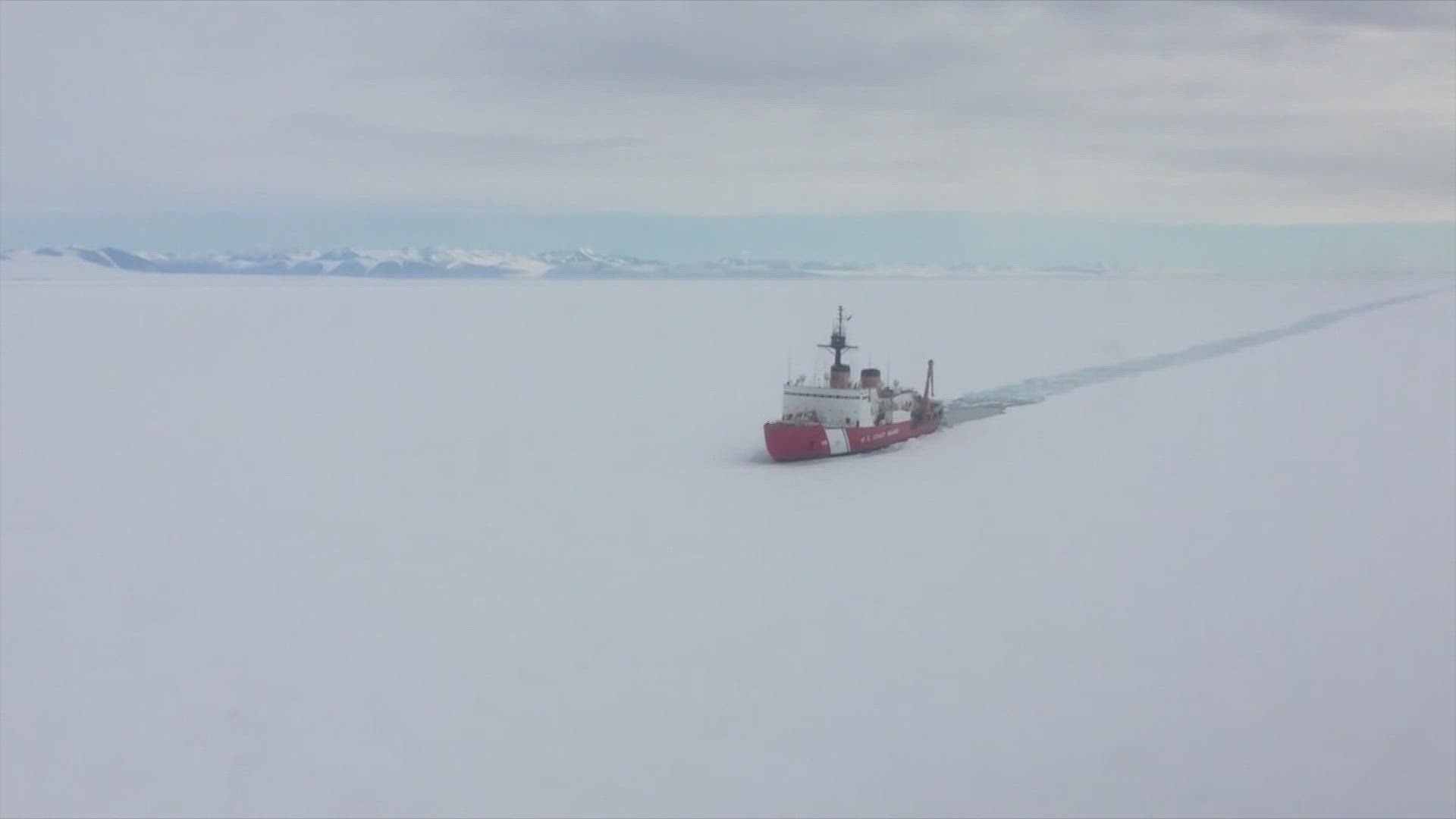The image depicts an aerial view of an Arctic scene, featuring a lone tugboat navigating through ice-covered waters. The boat, predominantly red with a white superstructure, is making a path through the icy landscape, leaving a clear trail behind it. Two brown smokestacks and an antenna rise from the top of the vessel, which appears to be engaged in plowing through the thick ice and snow. The backdrop includes towering mountains shrouded in clouds, with a narrow strip of blue sky visible between the ocean and the mountains, adding depth to the scene. The overall atmosphere of the image conveys extreme cold, with the predominant colors being white, blue, and red. The tugboat, heading from the right side of the image to the left, stands out as the main subject of this somewhat blurry yet striking Arctic photograph.